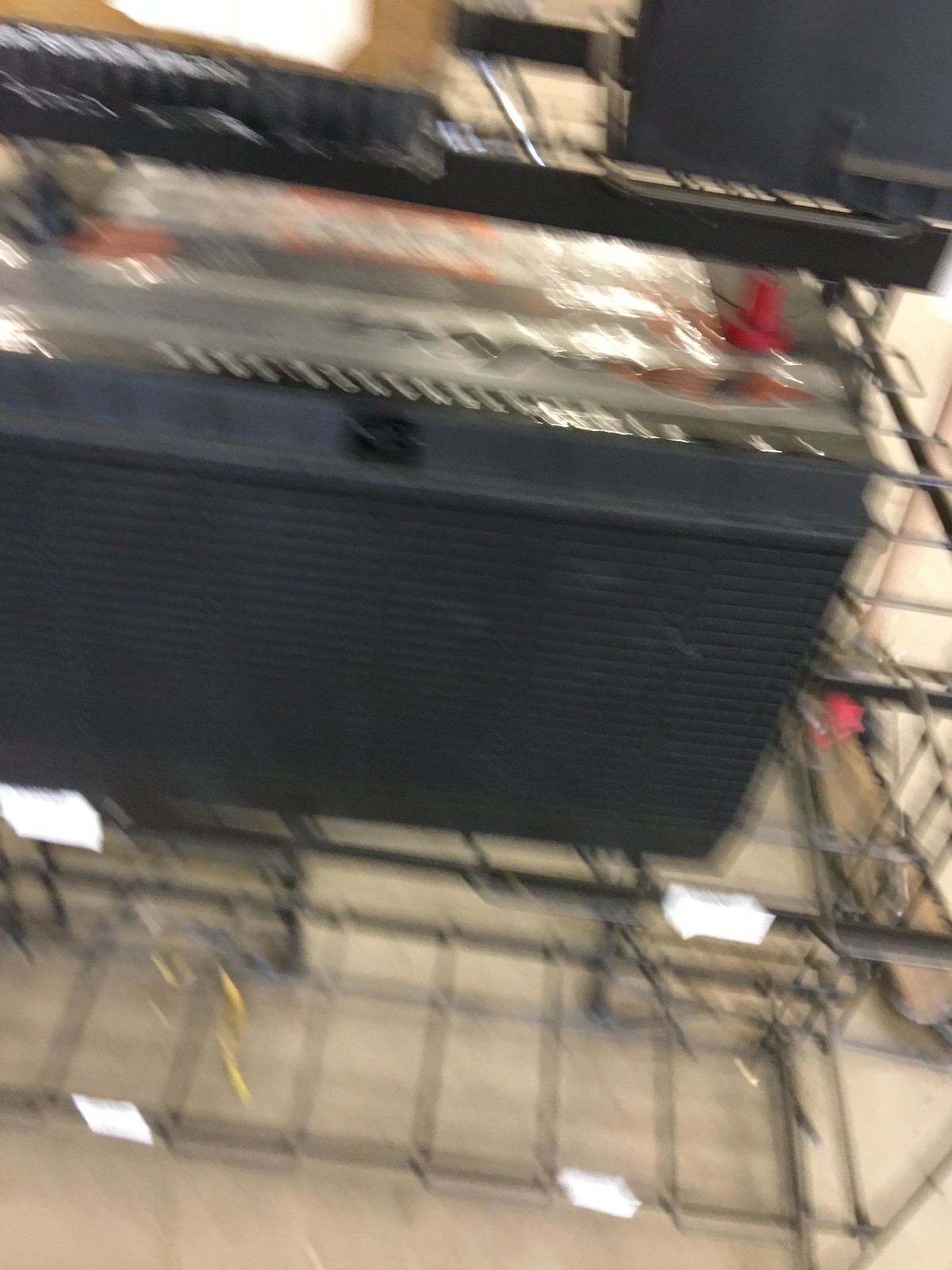This is a very blurry color photograph depicting a scene likely indoors. At the center, a black item is placed on a metal wire shelving unit that somewhat resembles a television or other electronic equipment rack. The black item might be a car battery or an electronic device like a boom box or the back of a television set, as indicated by its black metal casing and corrugated slots on the back, along with a couple of red knobs or extruded plastic pieces atop it. The shelving unit and the black plastic container appear to be situated on a light beige or brown floor, with some wires or debris scattered around, adding to the sense of disarray. The photograph does not contain any people, writing, plants, or buildings, and its vertical orientation emphasizes its length over its width. Additional items and potential background structures are indistinguishable due to the extreme blurriness of the image. This vague and indistinct setting hints at a storage area, possibly a warehouse or a space with leftover retail stock.